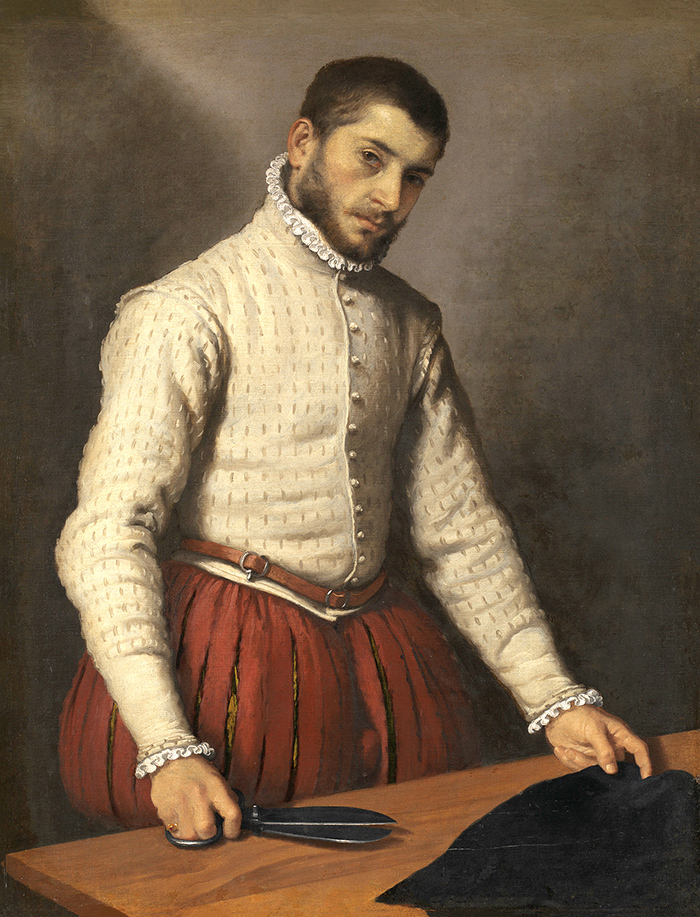In this detailed painting, an old-time tailor is captured in the midst of his craft. The background features a gradient with a darker brown hue on the left, transitioning to a thinner, lighter gray on the right. The tailor, an older gentleman with a beard and mustache, stands behind a sturdy brown wooden table. He holds a pair of large shears in his right hand, while his left hand delicately grips a piece of black fabric. His attire suggests a period from centuries past, possibly the Renaissance. He is dressed in a cream-colored, long-sleeved button-down shirt adorned with ruffled collars and cuffs. The buttons run in a precise vertical line down the center. Over his shirt, he wears a reddish garment resembling a skirt or dress. The composition lacks any text, focusing solely on the tailor and his surroundings. The dominant colors in the artwork include brown, red, cream, white, and black, adding to the vintage and timeless feel of the scene.